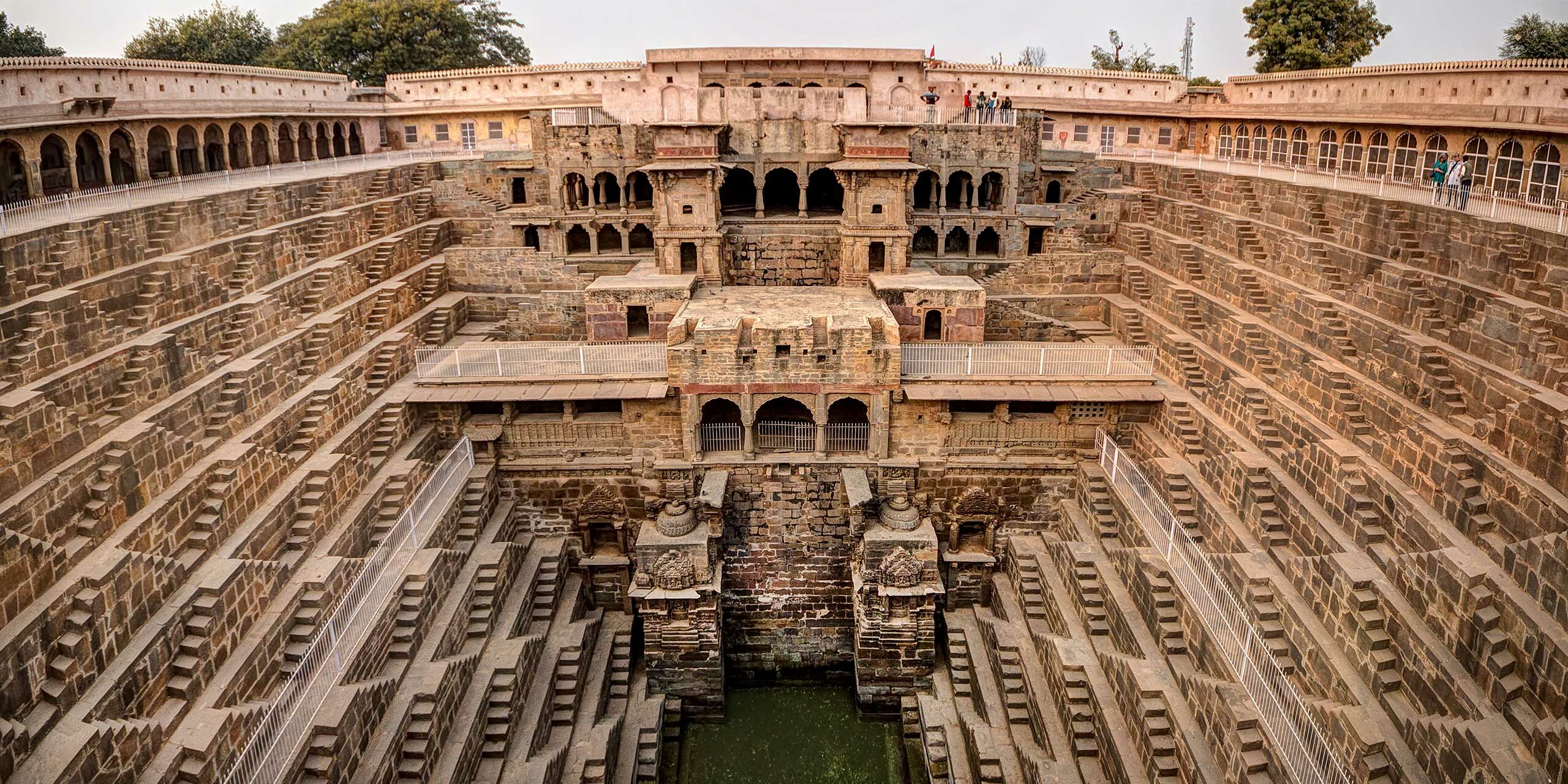This image depicts the panoramic view of a large, Colosseum-like stone amphitheater. The structure, made predominantly of aged beige and brown stones accented with stripes of red, features multiple descending rows of stairs and seating areas leading down to a central area that resembles a green field. This central area might serve as a body of water or sluice gate. The amphitheater is open-air, with no roof, and boasts beautifully crafted archways which allow light and movement through the area. Some sections appear to have modern additions, such as newer constructed stairs and railings that prohibit entry to certain parts of the structure. The top level of the amphitheater has people standing along the railing, indicating it might be a popular tourist destination. Adding to the scenic backdrop are trees situated above the structure, with the sky appearing to be blue but described as gray in spots. Notably, there are also designated areas, presumably for royalty, marked by white fences, and the entire setup tapers elegantly towards the center, enhancing its grand, arena-like ambiance.